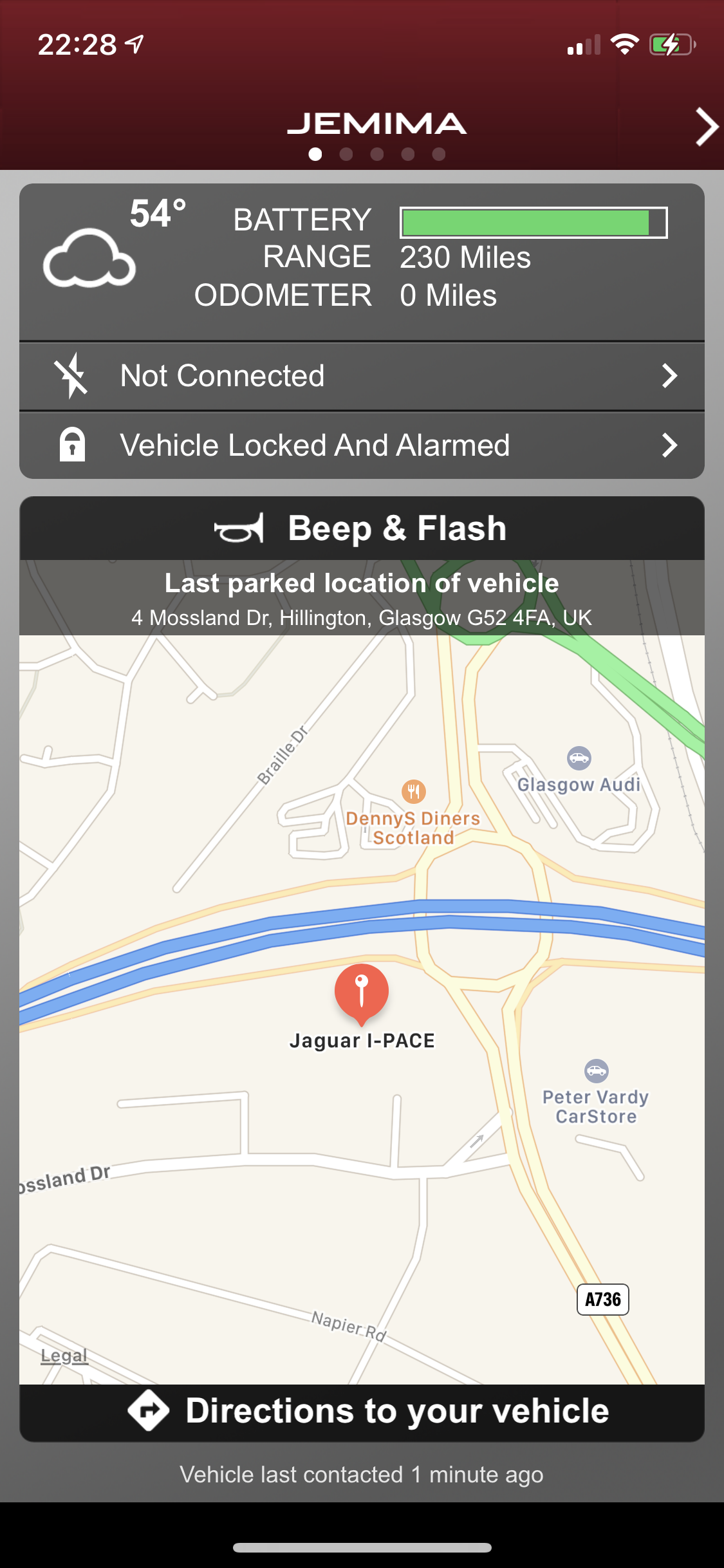This screenshot from a cell phone app provides a comprehensive view of a map and detailed vehicle information. The primary feature is a vertically oriented map, similar to Google Maps, with color-coded streets: a yellow map with blue marking a major road, a green highlighted road with a roundabout at the top, and various white streets labeled with their names. A dot indicates the location of a Jaguar I-PACE, signifying the user's position. At the map's bottom, there's a directive: "Directions to your vehicle," with a right-turn arrow, followed by "Vehicle last contacted one minute ago" in white text.

Above the map, the text reads "Last parked location of vehicle," providing the address: Mossland Drive, Hillington, Glasgow, G52 4FA, United Kingdom. Further up, there's an option "Beep and flash" with a horn icon for location signaling. A weather widget in the top left shows a temperature of 54°F with a cloud icon.

To the right is battery information: a nearly full green bar labeled "Battery," indicating a high charge level, possibly around 90%, followed by "Range: 230 miles" and "Odometer: 0 miles." Below these, there's a lightning bolt icon with a line through it and "Not connected," alongside a right-pointing caret. Another section beneath it shows a padlock icon labeled "Vehicle locked and alarmed," also with a right-pointing caret.

The top section displays "Jemima" in a futuristic font with five navigational dots below, the first one highlighted. The upper corners show the time (22:28 on the top left) and status icons for network signal, Wi-Fi, and battery charge on the top right.